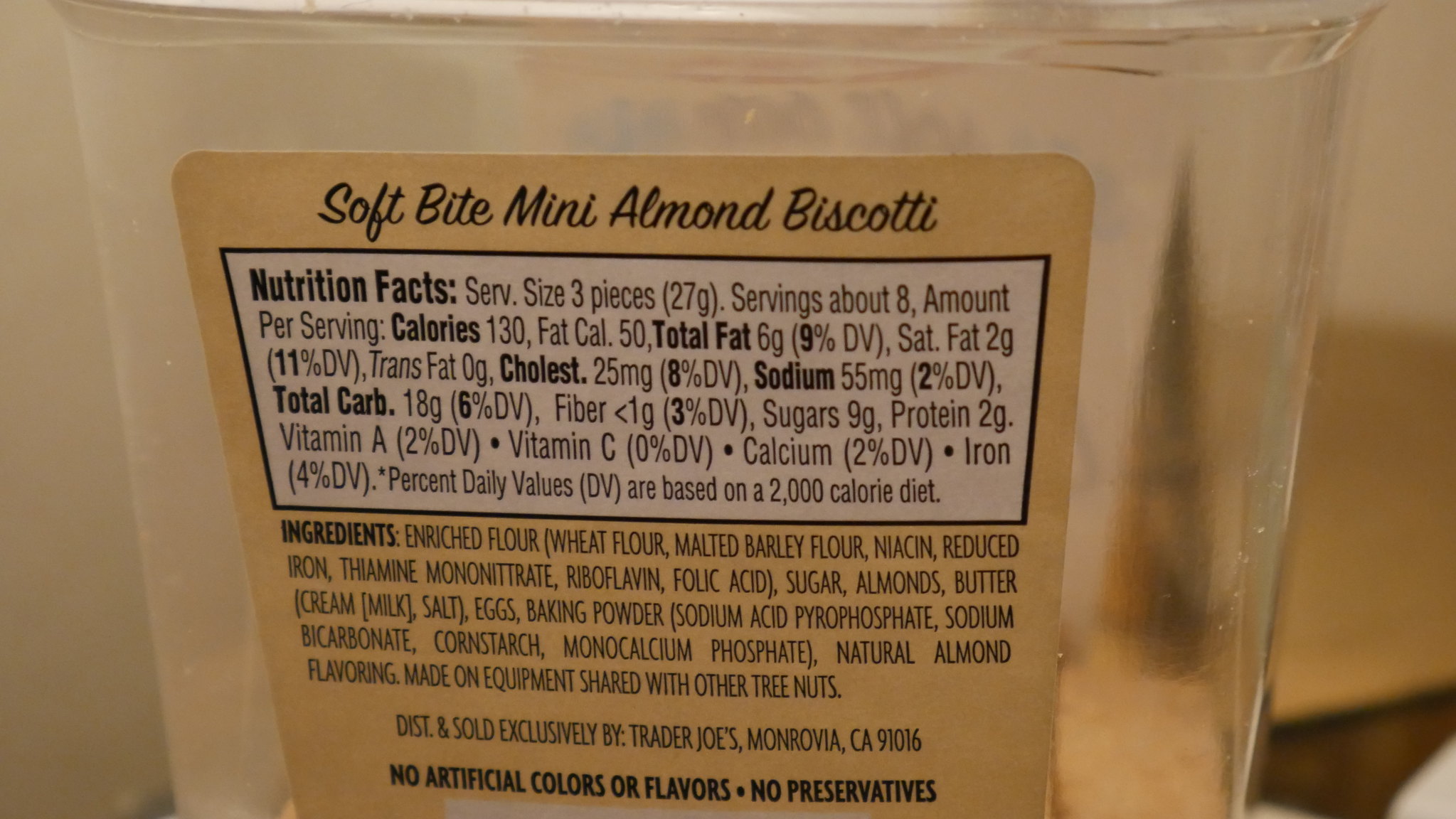Here is a detailed and polished caption for the image:

"This detailed image captures the back label of a product named 'Soft Bite Mini Almond Biscotti' affixed to a transparent or translucent jar. Inside the jar, a few flat biscotti biscuits are visible at the bottom. The back label prominently features a white box containing comprehensive nutrition facts, accompanied by a detailed list of ingredients located beneath it. Following the ingredient list, there is a distribution statement indicating that the product is distributed by Trader Joe's in Monrovia, California. The product proudly states that it contains no artificial colors, flavors, or preservatives. The ingredient list begins with enriched wheat flour and concludes with a note mentioning that the biscotti are produced on equipment that is shared with nuts."